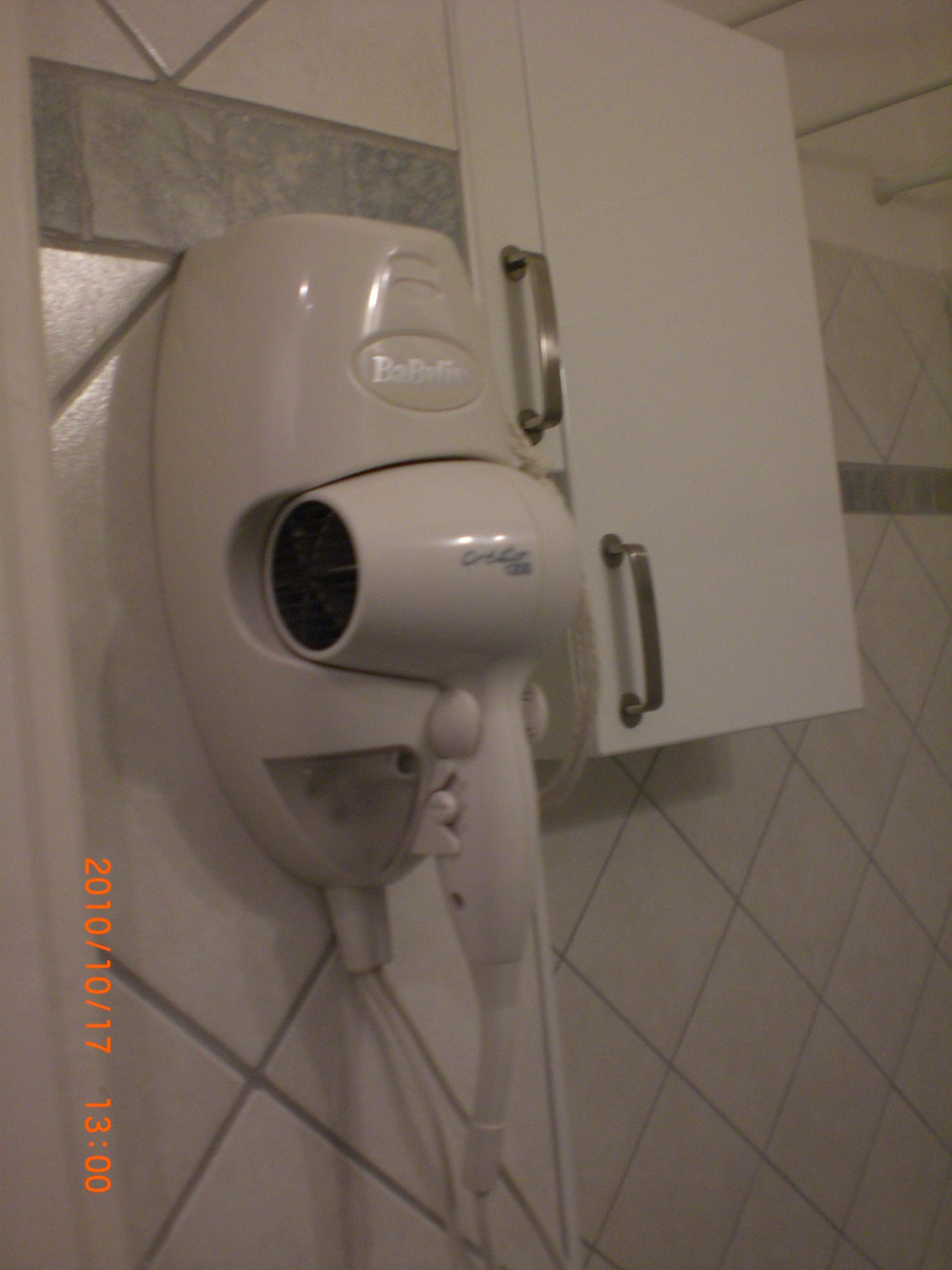This image is a detailed snapshot of a pristine bathroom, possibly in a hotel, given the organized and functional layout typical of such environments. The bathroom walls are adorned with off-white tiles arranged diagonally, forming diamond shapes, with a brown tile stripe running near the top. The tiling appears very clean and pristine. Mounted on the wall is a small, off-white hairdryer nestled in a dedicated wall fixture marked with the partially readable silver lettering "BABYLI". The dryer is connected by a cord and lacks a diffuser, adhering to the minimalistic aesthetic. To the right, there is a white cabinet fitted with sleek, silver aluminum handles, likely for storing bathroom essentials. The overall bright and well-lit atmosphere of the room adds to the impression of cleanliness. Additionally, a timestamp in orange on the image reads "2010-10-17 1300," marking the photo as taken on October 17, 2010, at 1 PM. The ceiling is also visible and appears to be white.